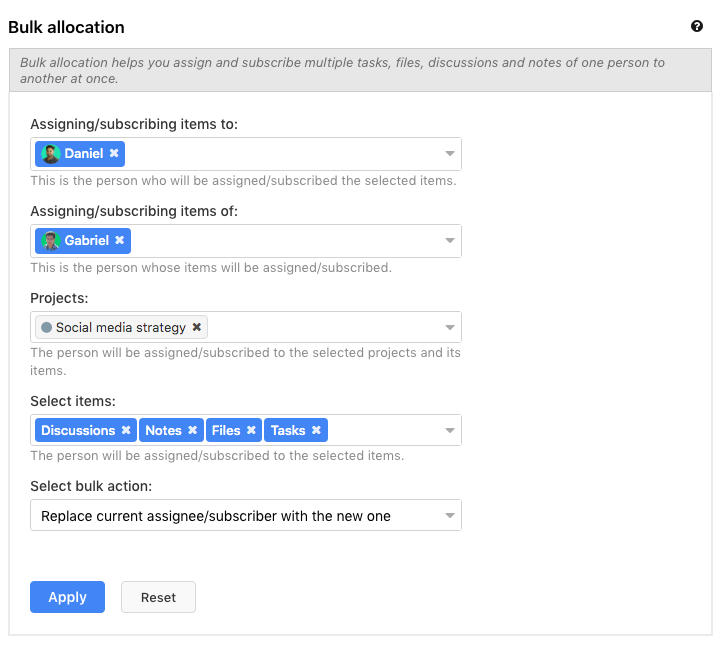Screenshot of the Bulk Allocation interface on a task management platform:

- **Background**: Solid white.
- **Upper Left Corner**: Black text reading "Bulk Allocation".
- **Upper Right Corner**: Black circle with a white question mark inside.
- **Below Header**: Gray banner with the text: "Bulk Allocation helps you assign and subscribe multiple task files, discussions, and notes of one person to another at once."
- **Main Interface** (white background with black text):
  - **Top Section**: 
    - "Assigning / Subscribing Items To"
    - Below it, a drop-down box containing a blue rectangle with the name "Daniel" and a white 'X' to the right.
  - **Middle Section**: 
    - "Assigning / Subscribing Items Of"
    - Below it, a drop-down box containing the name "Gabriel".
    - "Projects"
    - Below it, a drop-down box containing "Social Media Strategy" in a white rectangular box.
    - "Select Items"
    - Below it, a drop-down box containing four blue rectangular boxes labeled "Discussion," "Notes," "Files," and "Tasks".
  - **Bottom Section**: 
    - "Select Bulk Action"
    - Below it, a drop-down box reading "Replace Current Assignee/Subscriber with the New One".
    - **Lower Left Corner**: 
      - Blue "Apply" button.
      - White "Reset" button.